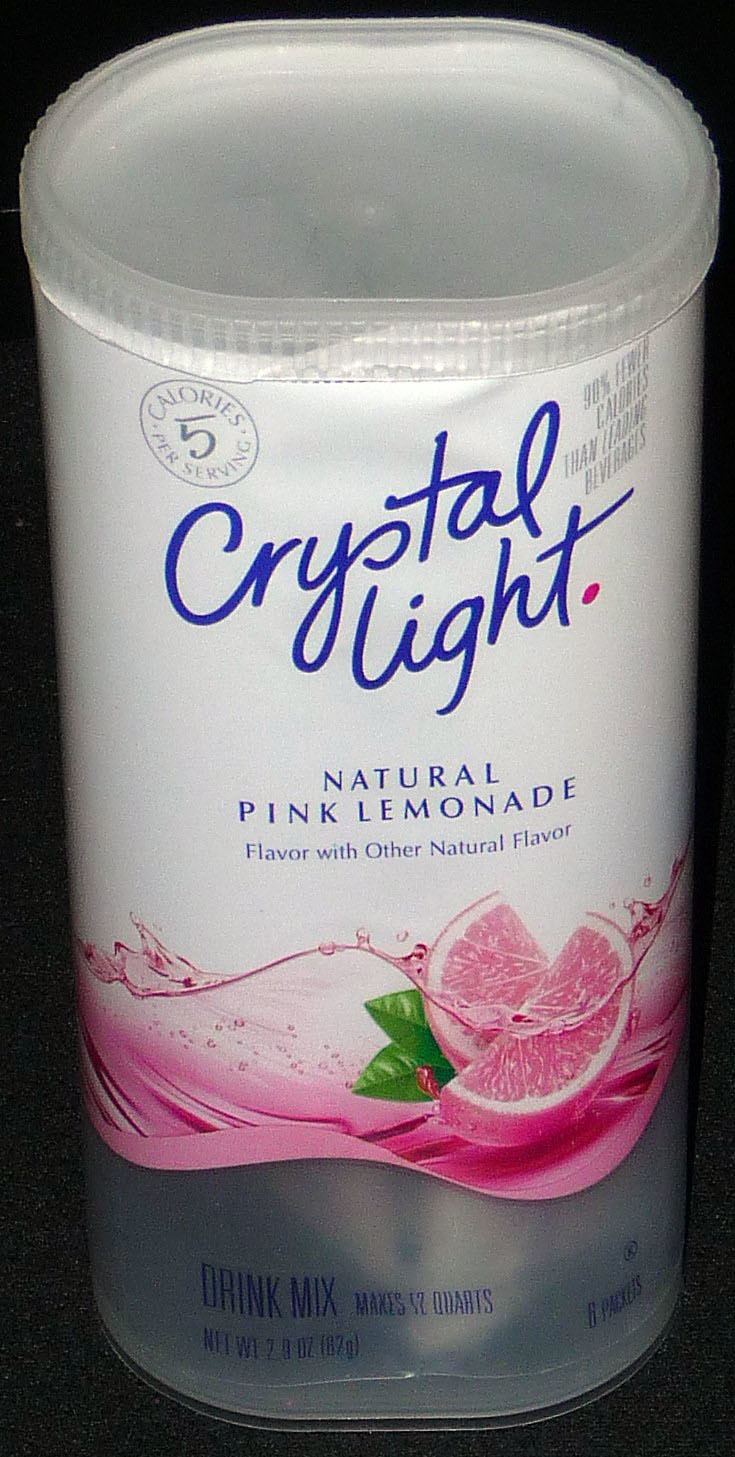The image is a vertically oriented and relatively narrow photograph of a Crystal Light Natural Pink Lemonade container. Captured from a top-down perspective, the container appears foreshortened, making the top seem slightly wider than the bottom. The label is densely packed with text and imagery.

At the very top of the label, "Calories 5" is prominently displayed. The product name, "Crystal Light," is written in a blue, handwriting-style font. Below it, in smaller text, the flavor is described as "Natural Pink Lemonade Flavor with Other Natural Flavors."

Centrally, a vibrant, wavy image of a pink grapefruit slice accompanied by fresh mint leaves adds a splash of color and visual appeal. Towards the bottom of the translucent container, additional text states: “Drink Mix Makes 12 Quarts,” “Net Weight 2.9 ounces (87 grams),” and “8 packets,” indicating the product's quantity and preparation instructions. The container holds a powdered mix for making Crystal Light lemonade.